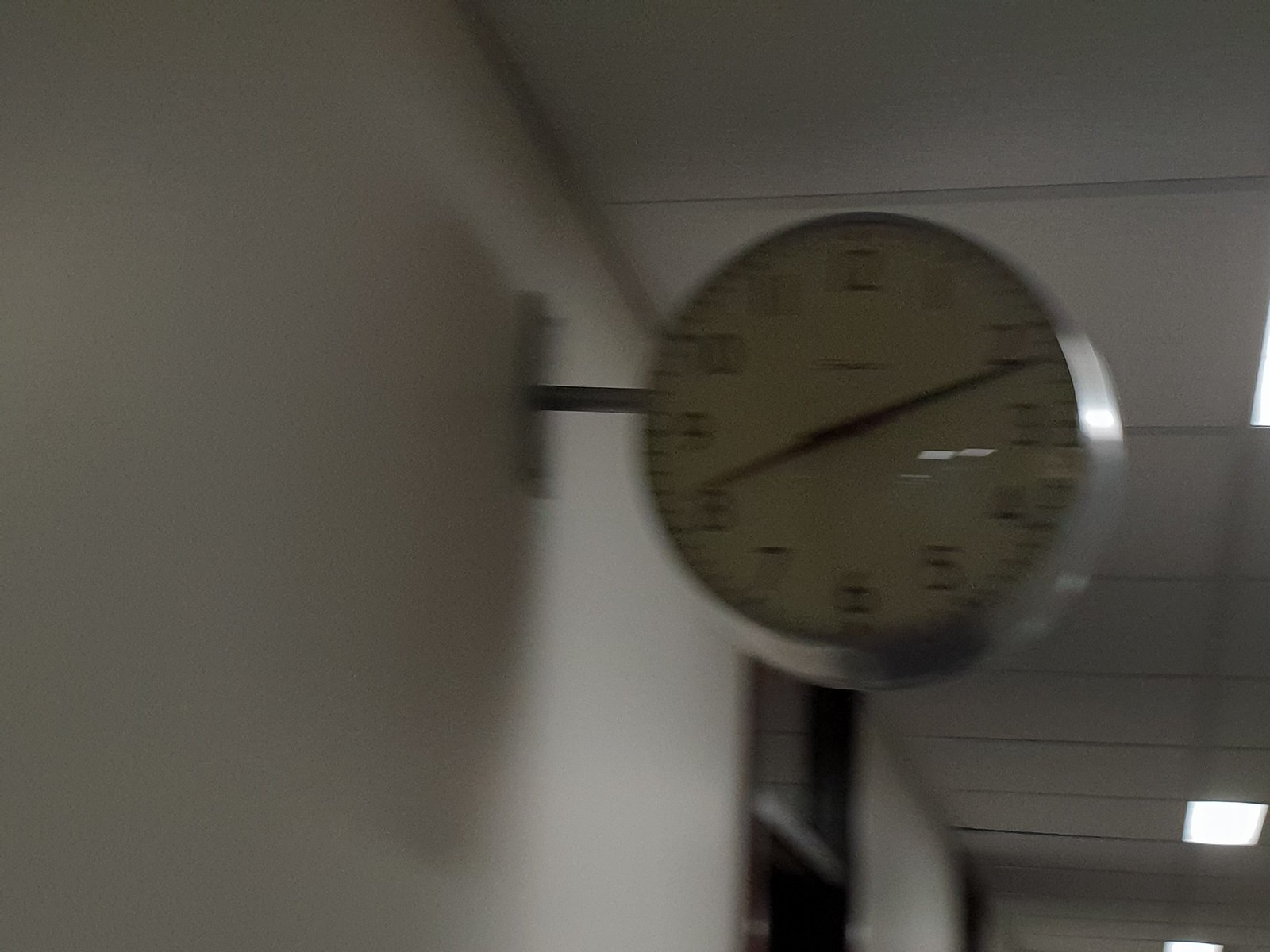The blurry image appears to capture an interior space, likely a school or an office building, featuring white walls with light gray shadows and a ceiling with darker gray lines separating asbestos tiles. Mounted high on the wall, a classic analog clock extends horizontally from a single metal rod, revealing two faces. The clock is outlined in silver with a white face, black numbers, and black hands, indicating a time of approximately 8:10. Below the clock, there is a door or window characterized by gray and black tones with a lighter gray stripe down the middle. The ceiling features several fluorescent lights, with three clearly visible on the right side, contributing to the shadows cast by the clock.